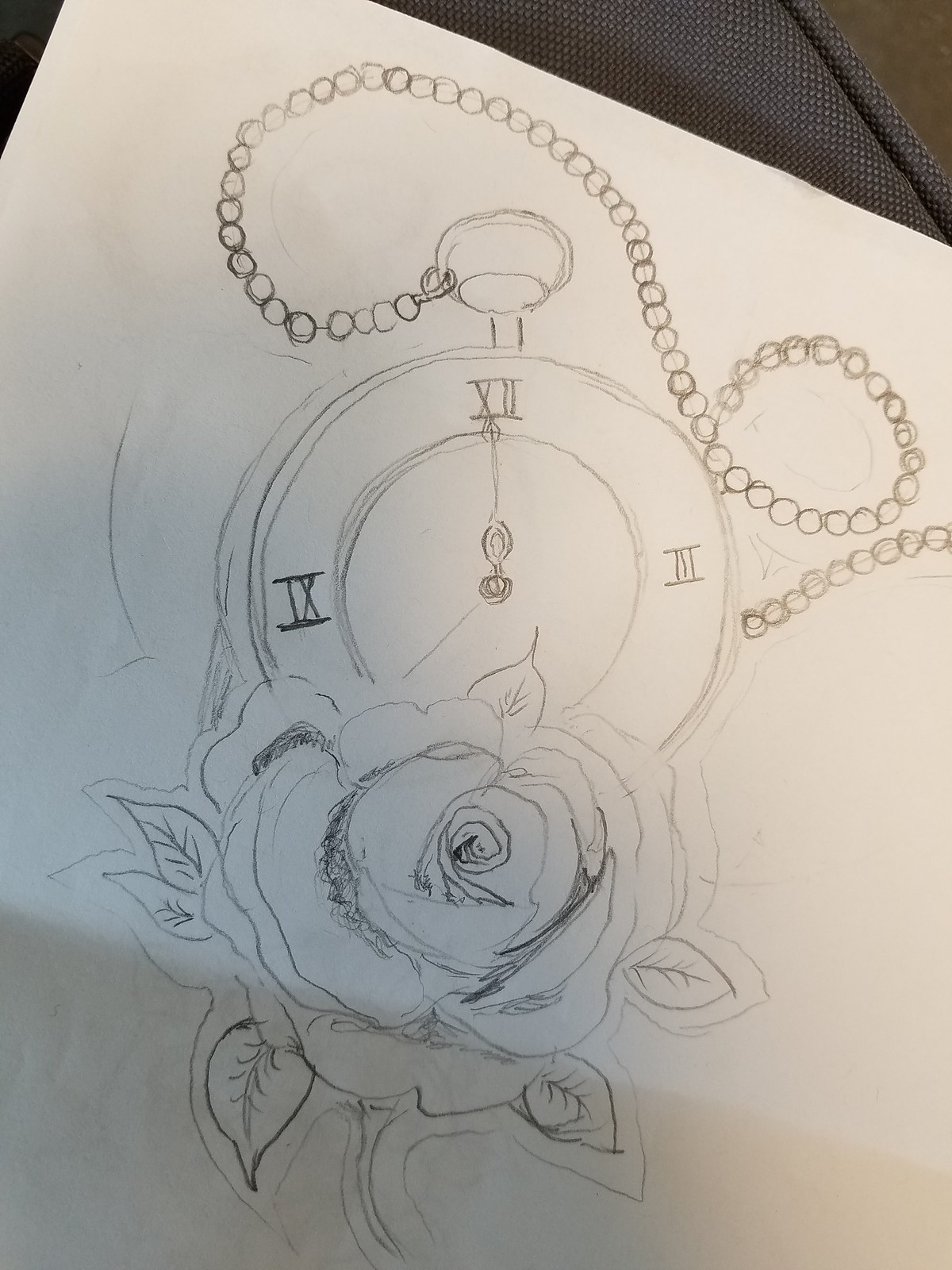This image captures a photograph of a detailed pencil drawing on white paper, situated within a sketchbook that's resting on a canvas chair. The drawing features a pocket watch displaying Roman numerals, with its hands positioned at either midnight or noon. Only a few numerals like XII, III, and IX are visible due to an intricately shaded rose positioned in front of it. The rose, with several leaves and a detailed stem, exhibits the most shading in the monochrome sketch. Extending from the top of the stopwatch is a chain, which curves around the drawing and stretches to the edges of the sketchbook page. The borders of the paper are slightly cut off, and a faint shadow is cast over the bottom of the image, enhancing the depth and dimension of the artwork.